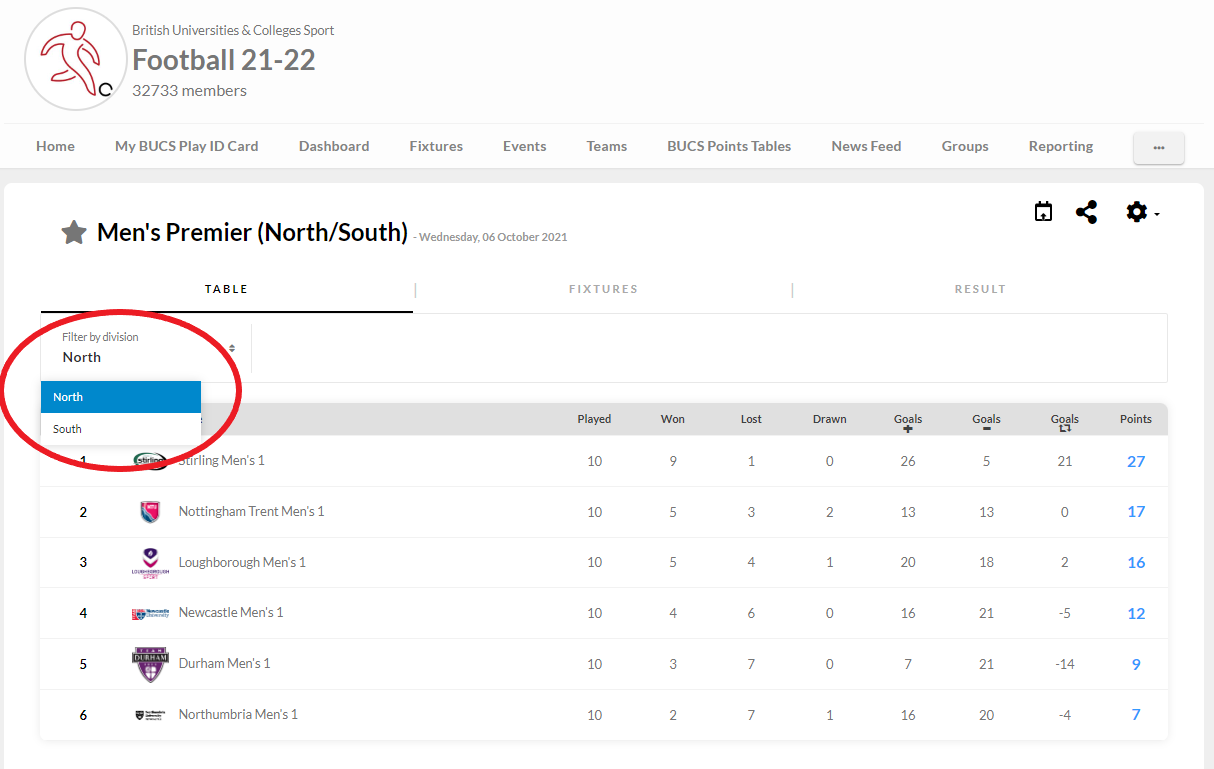In the top left corner of the image, an icon is displayed. Adjacent to it, within a circular emblem, a person is captured mid-kick with a soccer ball. Around this, text reads: "British University and College Sports Football 21/22" followed by "32,733 members."

Beneath this, a navigation row presents several clickable options including: Home, My BUCS, Play ID Card, Dashboard, Features, Events, Teams, BUCS Point Tables, Newsfeed, Groups, and Reporting. 

Below the navigation row, a prominent white rectangular area features a star icon. Accompanying this, in text, are the details: "Men's Premier North/South, Match Day: 16 October 2023." 

A section labeled "Table" is highlighted, suggesting its active status, with adjacent sections labeled "Results" and "Fixtures." Directly beneath this, a box labeled "Filter by Division" is visible, with a drop-down menu showing options for "North" and "South." The "North" option is highlighted in blue and encircled in red for emphasis.

Further down, a series of columns organizes information into structured categories.